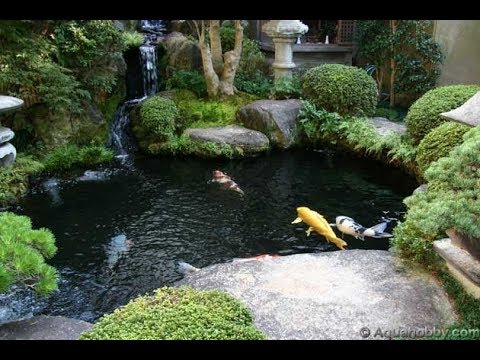A serene outdoor scene captures a small, picturesque pond at the center of the image. The water, appearing almost black, is dotted with large fish swimming near the surface, including a striking yellow one and a white-and-gray fish. The pond is encircled by large stones and meticulously manicured bushes, accentuating the verdant greenery that frames the scene. In the foreground, a sizable rock nestles among the greenery on both the left and right sides. Rounded, well-maintained shrubs add to the orderly beauty of the setting. In the background, a tree trunk stands tall, contributing to the lush surroundings, while a partially visible building with a window and a gray outer wall occupy the upper middle and right sections of the image, respectively. The composition is bookended by thin black horizontal bands at the top and bottom, adding a subtle framing to this tranquil garden tableau.